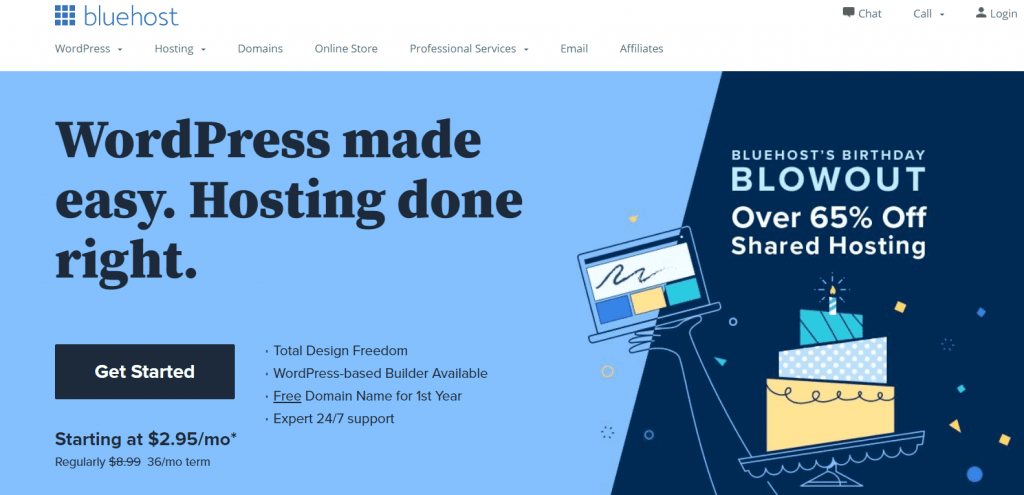**Screenshot of a Blue Host Web Page**

The top left corner of the screenshot features the Blue Host logo enclosed within blue boxes. Adjacent to the logo, on the right, are the options: "Chat," "Call," and "Login." Beneath these, a navigation bar lists various sections: "WordPress," "Hosting," "Domains," "Online Store," "Professional Services," "Email," and "Affiliates."

Central to the screenshot, the primary image showcases a celebratory theme. The backdrop of the image is a dark blue, decorated with an illustration of a cake that's whimsically tilted as if falling, accompanied by a hand holding a laptop. Above the cake, bold text announces the "Blue Host Birthday Blowout," promoting over 65% off on shared hosting. Confetti is scattered around to emphasize the festive atmosphere.

To the right of this primary section, a lighter blue background transitions sharply. Within this area, a headline reads, "WordPress Made Easy, Hosting Done Right." Directly below, a black button with white text urges viewers to "Get Started," followed by a pricing detail: "Starting at $2.95 a month, regularly $8.99, 36-month term." Adjacent to this, a bulleted list highlights key features: "Total Design Freedom," "WordPress-Based Builder Available," "Free Domain Name," and "Expert 24/7 Support."

Additionally, the screenshot contains arrows directing attention downwards next to the menu items "WordPress," "Hosting," "Professional Services," and "Call."

This comprehensive description mirrors the full layout and messaging observed in the Blue Host webpage screenshot.